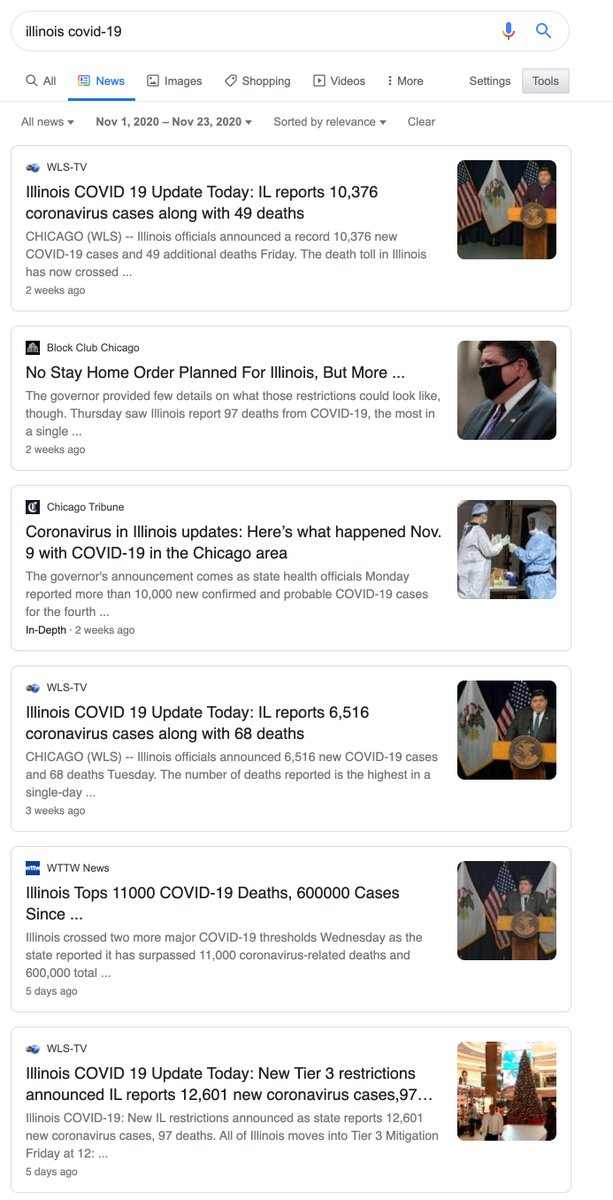The image displays a Google search results page focused on "Illinois COVID-19." At the top, the search query "Illinois COVID-19" is prominently displayed. Below it, various articles are listed, each with a thumbnail on the right side. 

1. The first article headline reads: "Illinois COVID-19 update today: Illinois reports 10,376 coronavirus cases along with 49 deaths." The accompanying text beneath the headline is too blurry to make out.
2. The second article states: "No stay-home order planned for Illinois," featuring a thumbnail of a man in a suit wearing a black face mask.
3. The third headline says: "Coronavirus and Illinois updates: Here’s what happened November 9th with COVID-19 in the Chicago area."
4. The fourth headline reports: "Illinois COVID-19 update today: Illinois reports 6,516 coronavirus cases along with 68 deaths."
5. The fifth article mentions: "Illinois topped 11,000 COVID-19 deaths, 600,000 cases since."

Overall, the search results highlight recent statistics and updates regarding COVID-19 in Illinois, including case counts, deaths, and government responses.